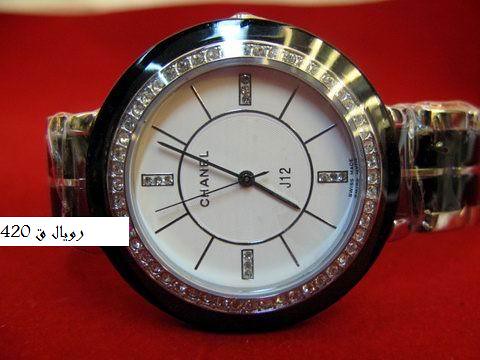This close-up color photograph showcases a beautifully ornate Chanel J12 wristwatch displayed on its side against a luxurious, red velvet-like background, giving it a sophisticated and high-end appearance. The watch, which needs to be rotated 90 degrees clockwise to view correctly, features a pristine white clock face. Markers at the 12, 3, 6, and 9 positions are rectangular and encrusted with small diamonds, while sleek black lines denote the other hours. The black watch hands indicate the time as 7:04.

The bezel is adorned with a continuous ring of diamonds encircling the glass face, further elevating its elegance. The watch band is primarily black, potentially made of leather or rubber, with detailed gold embroidery and a protective plastic wrap hinting at its new, unworn condition. A white rectangle overlapping the left side of the image displays the number "420" and Arabic writing, possibly indicating pricing or the model number for an online sale.

This photograph meticulously captures the luxury and craftsmanship of the Chanel J12 wristwatch as a coveted item, likely showcased for an opulent jewelry shop or high-end retail website.